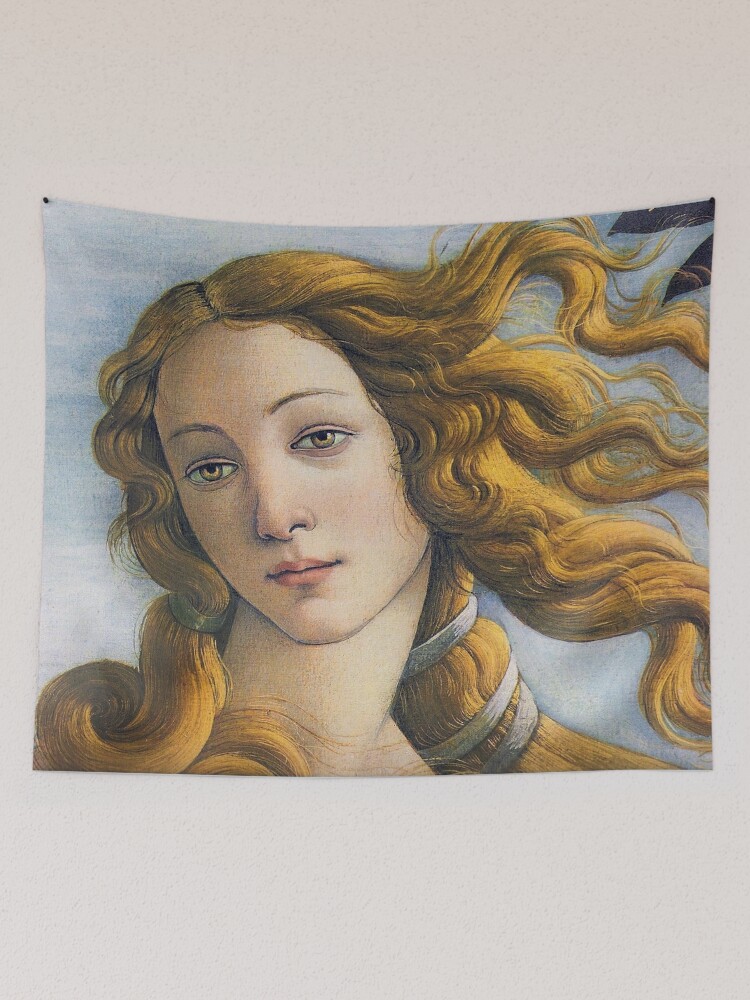This photograph showcases a detailed image of a woman on a piece of stretched fabric, secured to a white wall using four dark blue pins, placed in the upper left and right corners. The fabric displays a vivid painting with a cyan blue background and splotches of white near the woman's head.

The woman, possibly inspired by mythological figures such as Venus or a Viking princess, has flowing, curly hair cascading beyond her shoulders, bound with silver rings—three on the right side and one on the left. Her thick, lustrous hair features deep brown as the primary color with orange highlights and golden tones accentuating its vibrancy. Her head is inclined slightly to the left, exhibiting an expression of serene contemplation with downcast brown eyes that reflect a golden hue beneath the pupils. She possesses a light, smooth complexion with fine, brown eyebrows and a thin nose. The background features dark blue, leaf-like objects on the far right, and the painting is reminiscent of classical art themes, with subtle modern interpretations.

Overall, this captivating portrait merges elements of various historical styles, invoking imagery of myth and legend alongside contemporary artistic techniques.